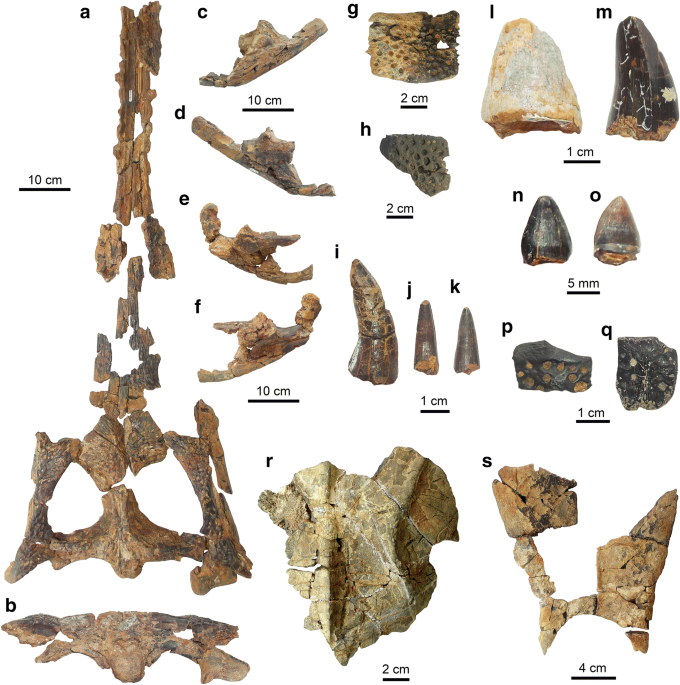This detailed image showcases a variety of fossilized animal bones, each labeled with letters from A to S and specific measurements. The bones, appearing brown and black, suggest they have undergone fossilization. Notably, the measurements are underlined: A, C, and F are marked at 10 cm, G and H at 2 cm, L, I, and P at 1 cm, R at 2 cm, and S at 4 cm. Some bones resemble undefined shapes, potentially resembling parts like hip bones. Towards the upper right corner, there's a distinctive black, arrow-shaped or tooth-like fossil marked with an 'M,' and next to it on the left, another similar but white and brown fossil marked with an 'L.' Both have a 1 cm measurement beneath them, consistent with the layout for the other fossil fragments. The image highlights the diversity and meticulous labeling of the bones, emphasizing their assorted sizes and the intriguing, fossilized appearance.